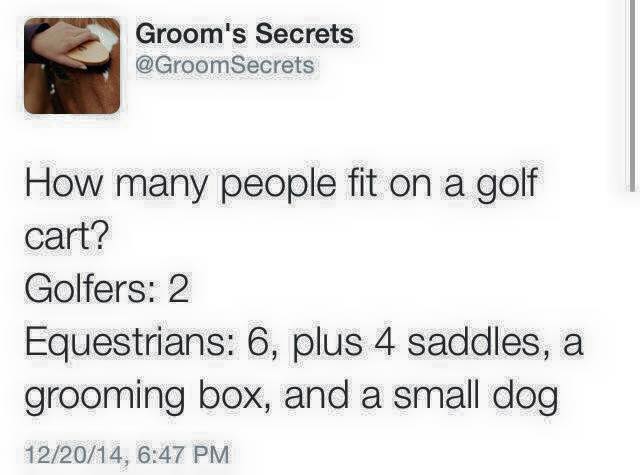This image captures a screenshot of a tweet from the now-older format of Twitter. The tweet, authored by Groom Secrets (@GroomSecrets), humorously compares the occupancy of a golf cart by golfers and equestrians. It reads: "How many people fit on a golf cart? Golfers: 2. Equestrians: 6, plus 4 saddles, a grooming box, and a small dog." The tweet was posted on December 20th, 2014 at 6:47 PM. Adjacent to the tweet, there’s a small, somewhat dark thumbnail image showing a left hand holding either a brush or a circular object with some foam underneath, suggestive of grooming or cleaning. The tweet playfully suggests that equestrians require more gear and space, adding a grooming box and a small dog to their count.